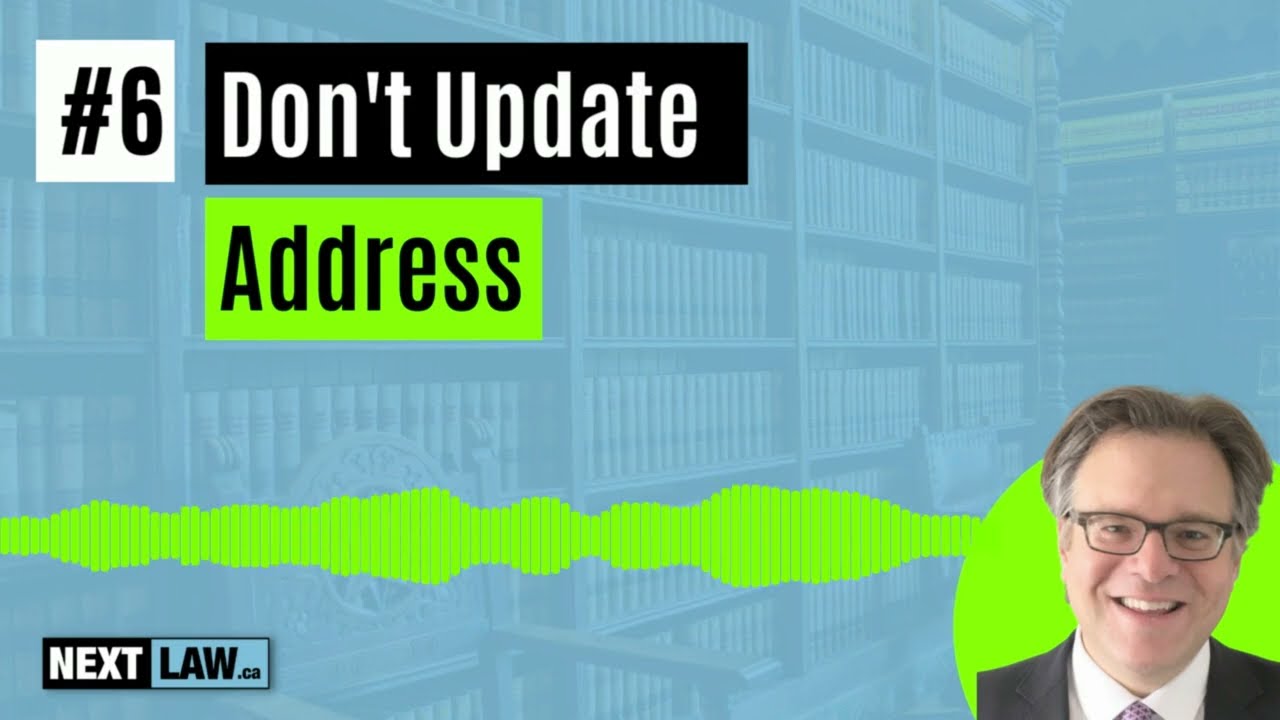The image appears to be a section of a PowerPoint slide or similar presentation, featuring a visually striking design and informative content. In the top left corner, a white square with the black number "6" is prominently visible above a black rectangle containing the words "Don't Update." Below this, a smaller green rectangle displays the word "Address" in black text. The background consists of a translucent blue overlay depicting rows of books, suggesting a library or law office setting.

Centrally and slightly to the right, a lime green circle encloses the smiling face of an older white man. He has light brown hair with hints of gray, wears dark-framed glasses, and is attired in a suit consisting of a black blazer, white shirt, and partially visible red tie. His image is cropped from the shoulders up, revealing his friendly expression and top teeth. Extending from the green circle are horizontal wavy lime green lines, which merge into a green voice bar consisting of vertical lines of varying lengths, reminiscent of audio levels.

At the bottom left of the slide, in a small black box with white text, the word "next" is displayed. Adjacent to it, "law.ca" is written in black text within a blue rectangle, forming the web address "nextlaw.ca." This detailed and visually engaging slide conveys point number six of the presentation.